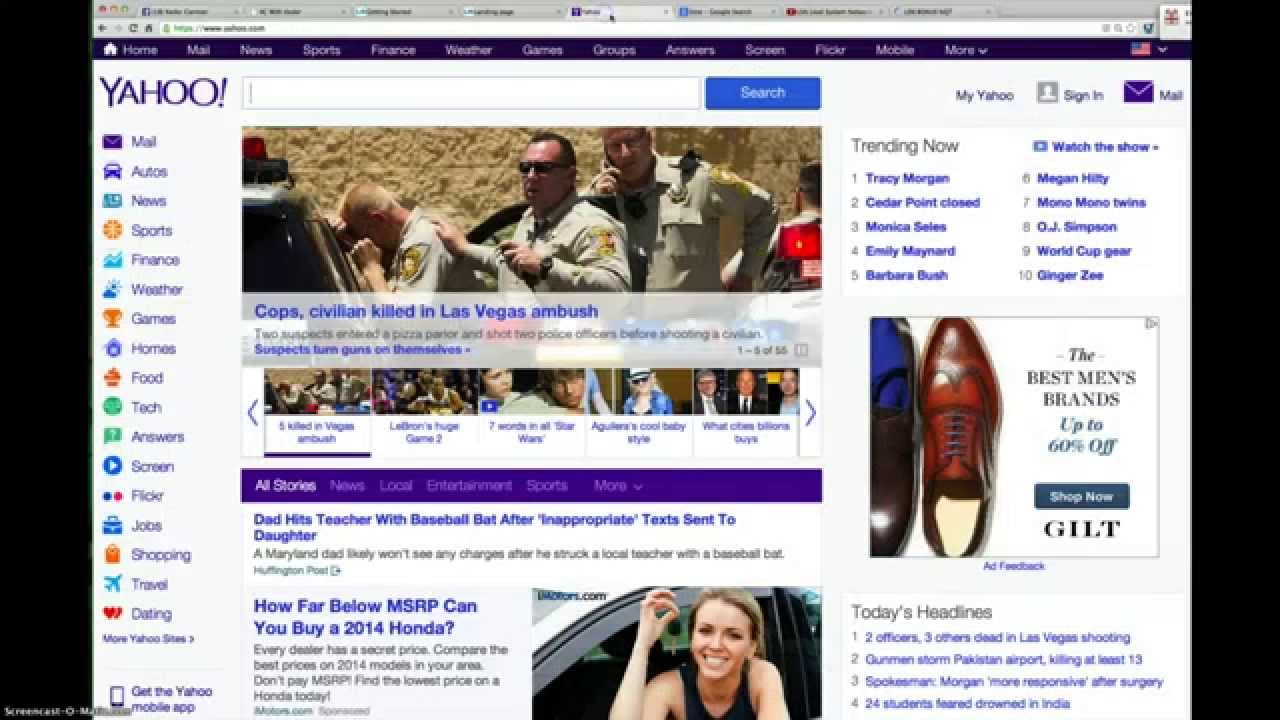This detailed caption offers a vivid description of the screenshot taken from an old Yahoo search engine webpage:

"A screenshot captures a crowded browser window with multiple tabs open. The highlighted tab displays a vintage Yahoo search engine page. The header of the webpage is distinctly purple, iconic of Yahoo's early design. At the top navigation bar lie various links including Home, Mail, News, Sports, Finance, Weather, Games, Groups, Answers, Screen, Flickr, and Mobile, with additional links available under a 'More' dropdown.

This is the landing page of the Yahoo search engine. The Yahoo logo, also in purple, is prominently positioned in the top left corner, adjacent to a search bar with a blue search button. Further along the same row are options for 'My Yahoo,' sign-in, and a mail icon.

Dominating the main content area is an article featuring three police officers in beige uniforms. One officer, appearing to grieve, is leaning against a patrol car. The headline of the article reads, 'Cops, Civilians Killed in Las Vegas Ambush.' Below this section, there are photo and video reels offering more visual content.

On the left sidebar, a list of Yahoo features is presented, each accompanied by an icon. Categories include Maps, Auto, News, Sports, Finance, Weather, Games, Homes, Food, Tech, Jobs, Shopping, Travel, and Dating.

On the right side of the page is a promotional banner titled, 'The Best Men's Brands from Gilt.' It pictures two polished dress shoes on a white background, featuring a green 'Shop Now' button and text proclaiming 'Up to 60% Off.'"